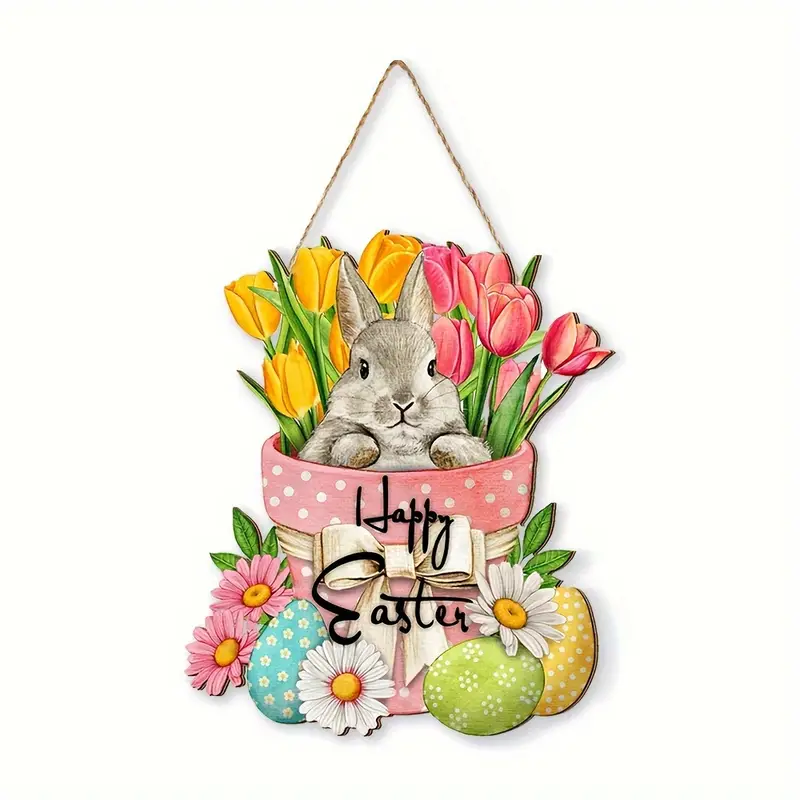This image portrays an artwork, potentially a drawing or digital art, of a playful and festive scene centered around a pink flower pot adorned with white polka dots and a white ribbon tied in a bow. In the middle of the pot, bold black letters spell out "Happy Easter." Sitting inside the pot is an adorable gray and white bunny with its ears perked up and front paws resting on the pot's edge, gazing outward. Surrounding the bunny inside the pot are vibrant yellow and pink tulips with lush green leaves and stems. The pot appears to be hanging from a thin thread or twine, suggesting it can be displayed as a decorative item. Below the pot, two pink daisies with yellow centers and green leaves frame the scene, accompanied by a trio of colorful Easter eggs decorated with floral patterns: a bright green egg with white flowers, a yellow egg with white polka dots, and a bright blue egg with daisies. This cheerful composition captures the essence of Easter celebration with its whimsical elements and bright, festive colors.